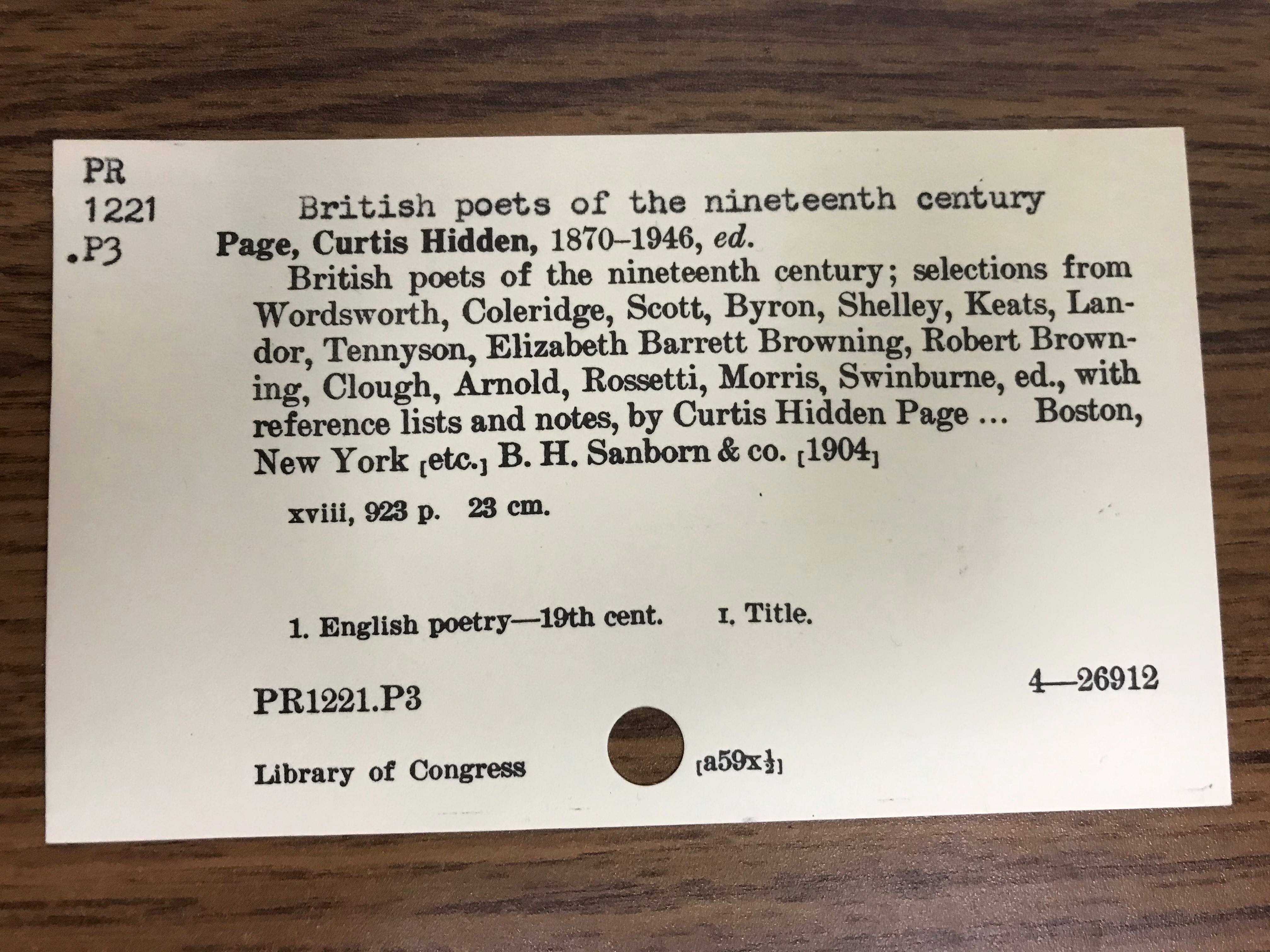The image features a typewritten library catalog card placed on a brown wooden table, viewed from above. The card appears to be from an old library index and contains detailed bibliographic information. In the top left corner, the classification code "PR1221.P3" is displayed. The main body of the card identifies the book as "British Poets of the 19th Century," edited by Curtis Hidden Page (1870-1946). It lists selections from poets including Wordsworth, Coleridge, Scott, Byron, Shelley, Keats, Landor, Tennyson, Elizabeth Barrett Browning, Robert Browning, Clough, Arnold, Rossetti, Morris, and Swinburne. The reference and notes are also provided by Curtis Hidden Page, and the publication details include Boston, New York, B.H. Sanborn & Co., 1904. Additional details such as "XVIII, 923 pages, 23 cm" and "Library of Congress" are noted at the bottom, along with a small hole punch near the center of the card.